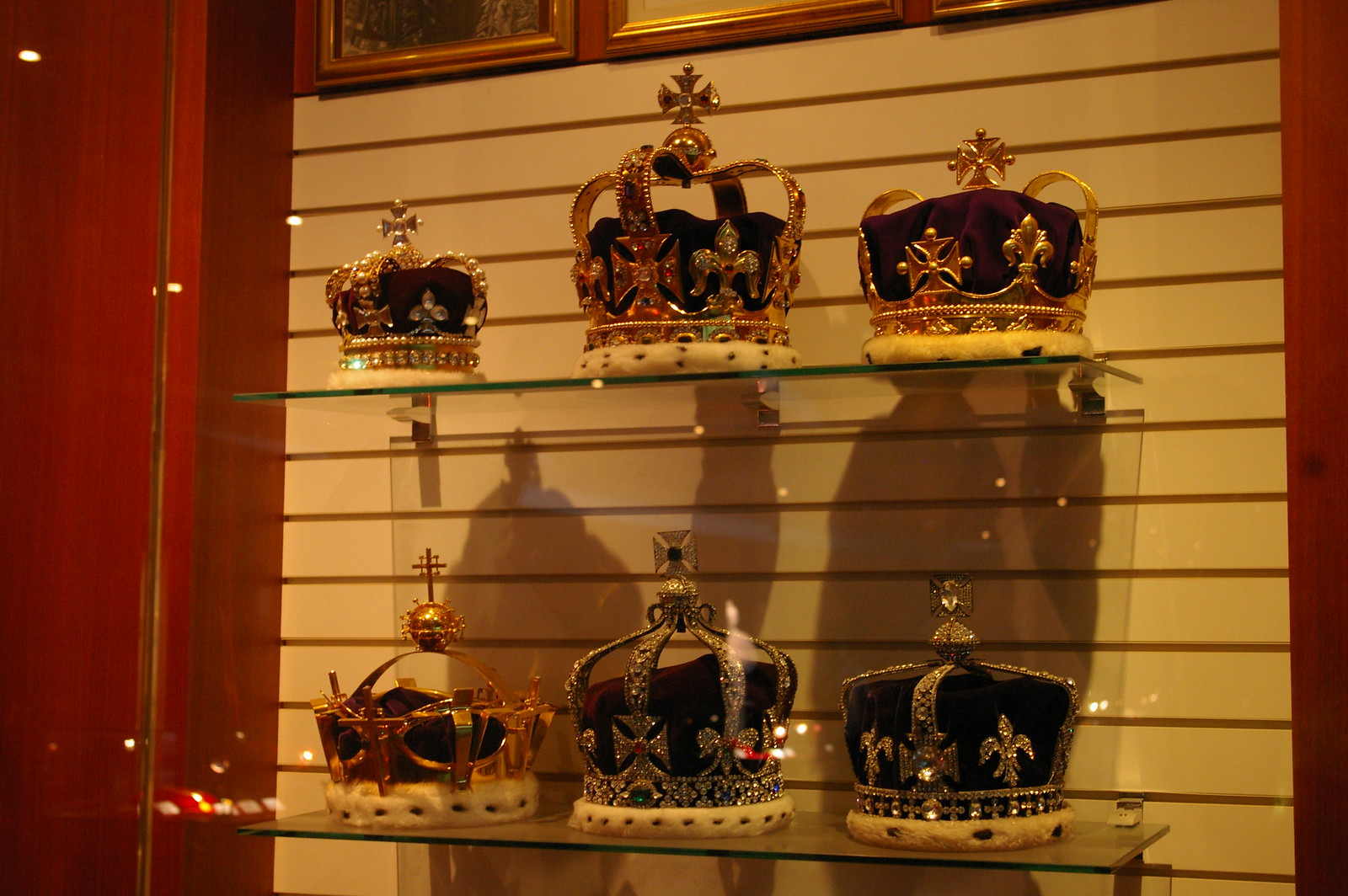This color photograph captures a detailed display case placed against a sliding section of a yellow-tinted wall, bordered by a reddish-brown outline. The display case, positioned centrally, contains two glass shelves, each showcasing three ornate crowns. Against the white backdrop within the case, these regal crowns exude an air of sophistication and history.

On the top shelf, three crowns are presented, each intricately designed with purple velvet interiors and rimmed with ermine fur, white with black dots. The crowns feature golden bands and are topped with a combination of balls and Maltese crosses. The smallest crown, positioned to the left, includes dark blue fabric inside, a gold base, and a golden cross at the center. The largest crown, centrally positioned, mirrors the fabric and cross design but with more pronounced gold bands. The crown on the right stands out with its red fabric interior, adorned with gold crosses along the front.

The bottom shelf mirrors the top with three similar crowns, each showcasing dark red fabric interiors and topped with gold crosses. Each crown casts a shadow against the white backdrop and is consistently rimmed with white, fur-adorned gold bottoms.

To the left of the photograph, part of a dark brown wall is visible, and above the display case, the lower portions of three framed pictures can be seen, contributing to the regal ambiance. The photograph is devoid of text and people, allowing the detailed craftsmanship of the six crowns to be the focal point.